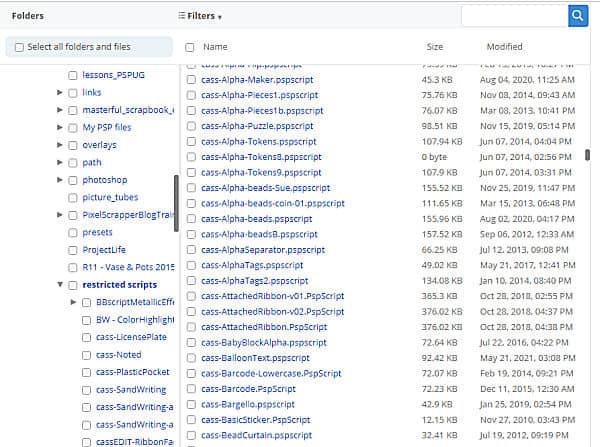This image is a low-resolution screenshot featuring a complex file management system with a variety of script files and folders. At the top of the screenshot, a series of gray bars are visible, along with folder and filter options.

On the left-hand side, a search bar is present, enabling users to select from a list of all folders and files. The searchable items are listed as follows:
- Lessons
- PSPUG
- Links
- Masterful Scrapbook
- My PSP Files
- Overlays
- Path
- Photoshop
- Picture Tubes
- Pixel Scrap or Blog Train
- Presets
- Project Life
- R11
- Basin Pots 2015
- Restricted Scripts

Under the Restricted Scripts section, there are further sub-items:
- bbscript
- meta
- italic effect
- bbw
- color highlights
- cast license plate
- cast noted
- cast plastic pocket
- cast sand writing
- cast edit ribbon file

The right-hand side of the screenshot predominantly displays various PSP scripts, many of which start with the prefix "cast-alpha-". Some of these scripts include:
- cast-alpha-maker
- cast-alpha-pieces1
- cast-alpha-beads-sue
- cast-alpha-beads
- cast-attached-ribbon

The modification dates for these scripts range from 2010 to 2019. Despite the low resolution, the individual letters and items can still be discerned, providing a detailed view of the numerous files and scripts available within this file management system.